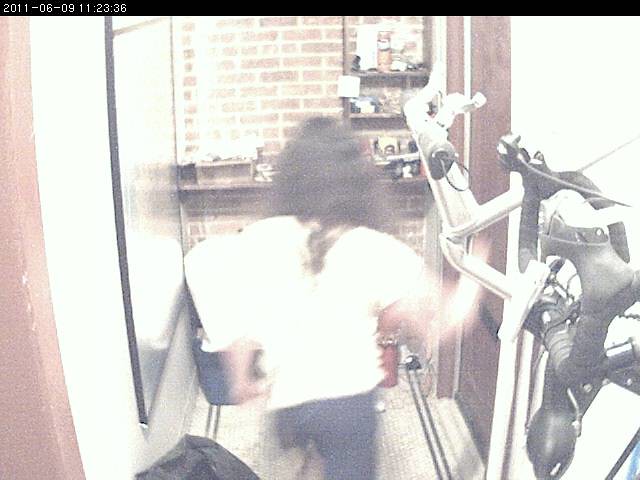In this security camera footage dated June 9, 2011, at 11:23:36, a person with long dark hair is captured standing in front of a brick wall. This individual is wearing a white short-sleeved shirt and dark pants. The background features a shelf mounted on the brick wall. To the left of the image, a robotic arm with various black, white, and silver components is visible. The floor is tiled, and on the right side, there is a black trash can partially in the frame, along with a glimpse of a wooden door frame. A black object is noticeable on the floor.